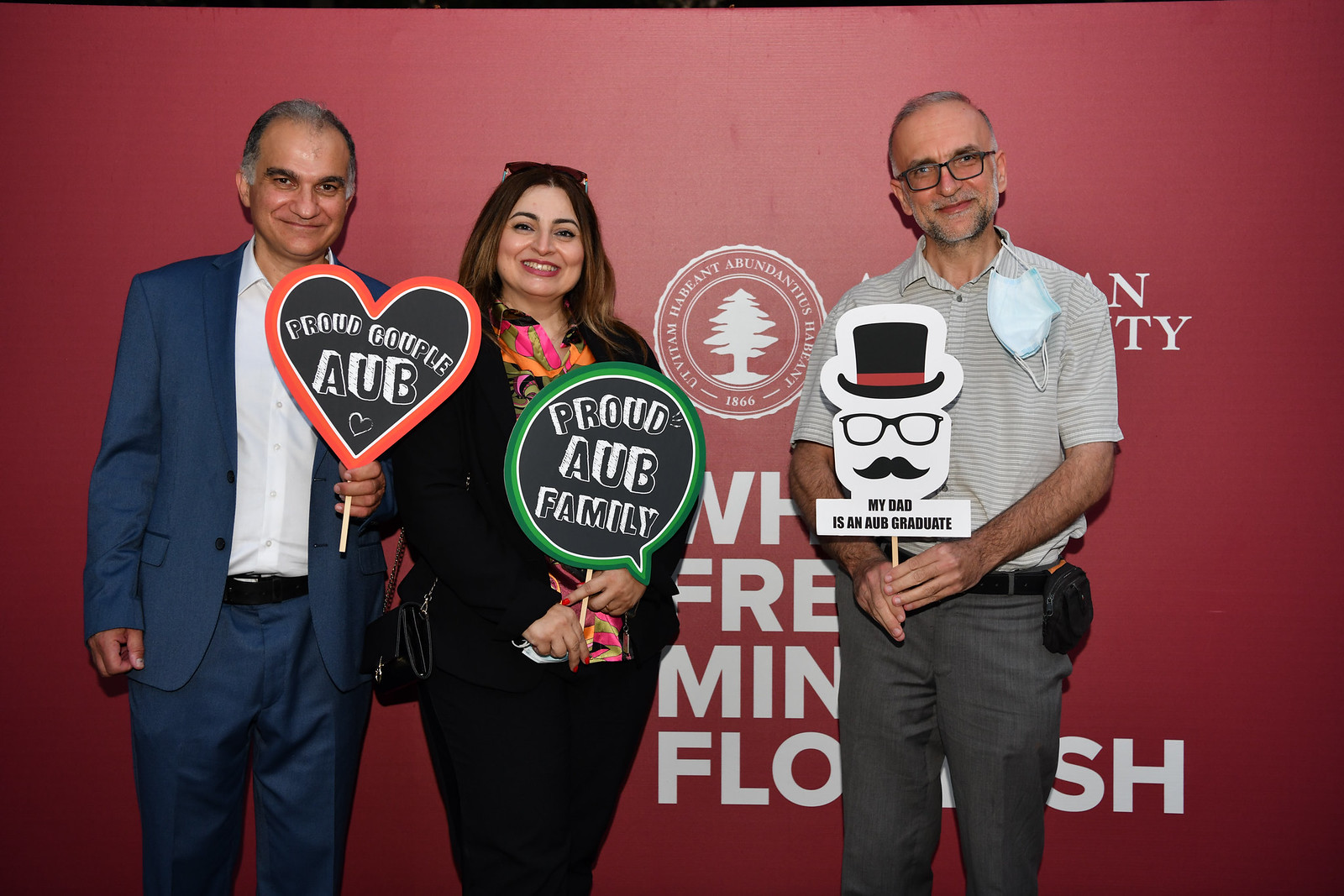In this photograph, three people are standing in front of a burgundy banner adorned with white text and a logo. On the left is a man with grayish hair, dressed in a blue suit with a white shirt and blue pants. He is smiling and holding a heart-shaped card outlined in red and black that reads "Proud Couple AUB." In the middle stands a woman with shoulder-length brown hair and sunglasses on her head, clad in a black coat and pants with a colorful shirt underneath. She too is smiling and holding a green speech bubble-shaped card that says "Proud AUB Family." On the right, a man wearing a white shirt with brown lines and gray pants is holding a sign shaped like a man's face with a hat, glasses, and mustache, inscribed with "My Dad is an AUB Graduate." Each person proudly displays their connection to AUB, forming a cohesive and joyful scene.